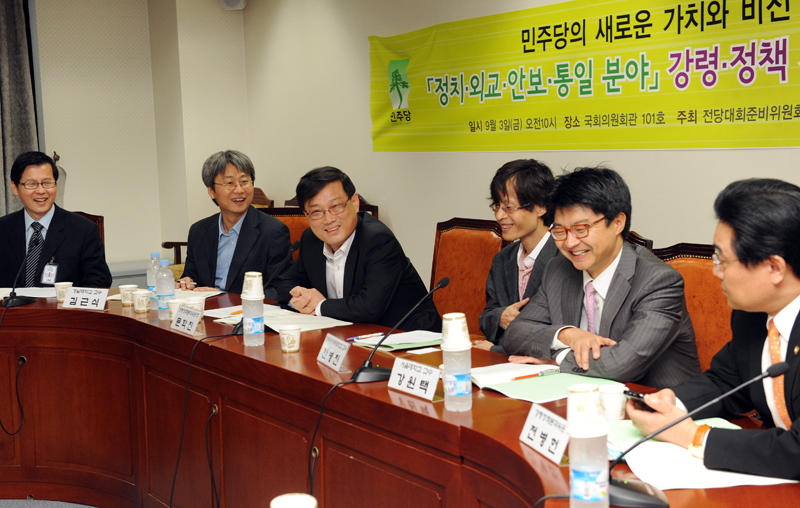The photograph captures an indoor scene of a formal meeting or committee session. Central to the image is a long, slightly curved wooden table, positioned from the lower right towards the center. Seated around this table are six men of Asian descent, each appearing relaxed and smiling. They are all dressed in suits, mostly dark in color, and all wearing glasses. Five of them have black hair, while the second man from the left has gray hair. In front of each man are nameplates, pencils, pens, bottles of water with small cups, and shared microphones that seem to serve every two individuals.

The background features a light-colored wall adorned with a prominent banner. This banner, which stretches from the upper right corner to the middle of the image, has a gold or yellow hue with text written in Korean, displaying characters in black, blue, and purple. The men are seated in orange leather chairs with wooden frames, collectively contributing to the formal yet cordial atmosphere of the setting.